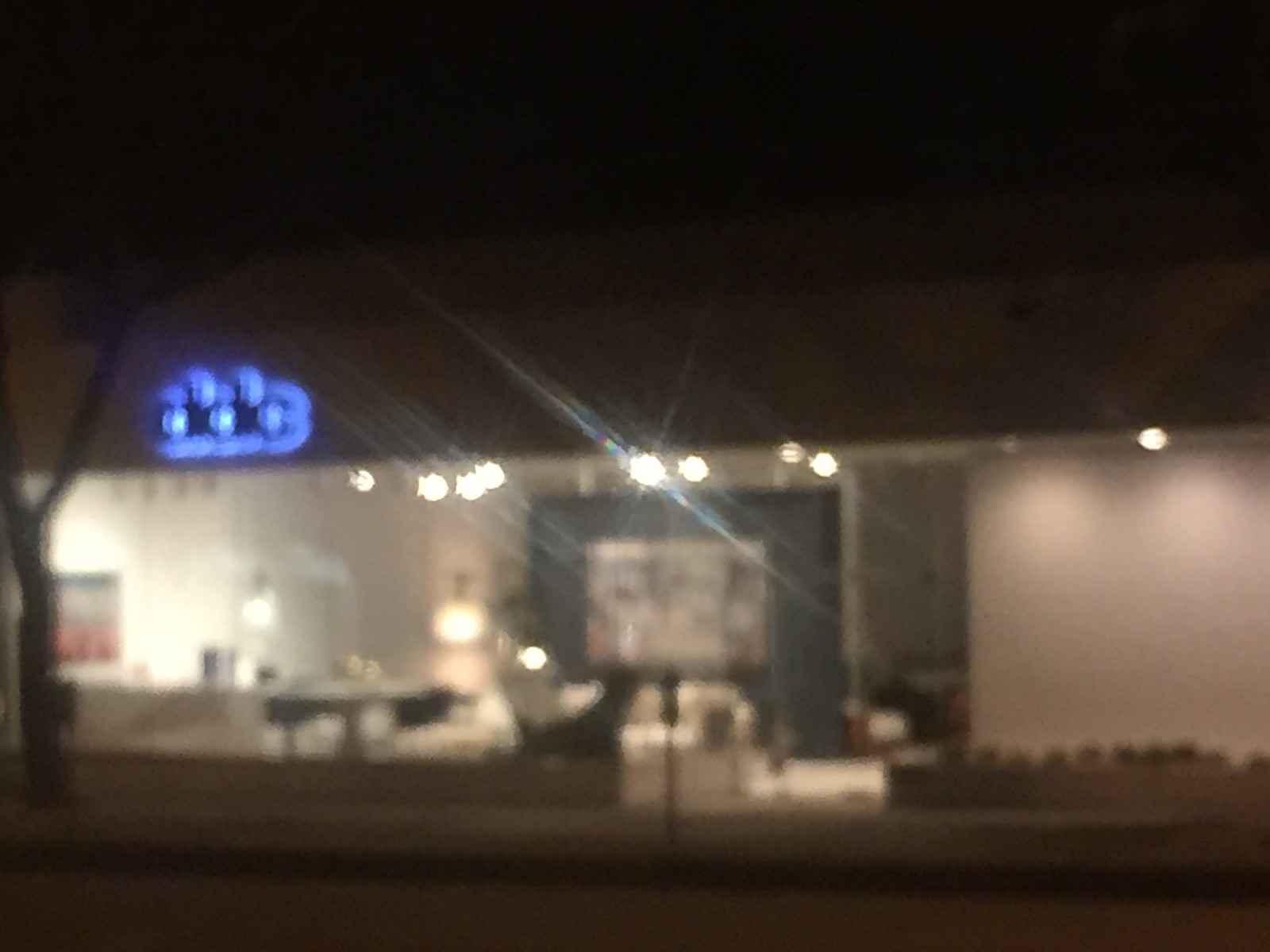The image depicts a dimly lit scene featuring the exterior and interior of a small, single-story building at night, possibly a store or restaurant. A black night sky forms the backdrop, contrasting with the building’s light gray roof and white exterior walls. The front of the building includes a glass façade, through which an assortment of furniture is visible, suggesting it might be a furniture store or a waiting room. The interior showcases white sofas, tables, and lamps, alongside a reception desk with a large colorful painting behind it. A blue neon sign at the building's top border displays letters, likely "DDC," although the text is blurred and difficult to decipher.

To the left of the frame, a silhouette of a tree is faintly visible, adding to the outdoor setting. The scene includes several empty parking spots equipped with meters, indicating that parking requires payment. The image quality is notably fuzzy, making finer details such as the precise letters on the neon sign and the design of the furniture appear grainy and indistinct. Furthermore, the building’s interior features a blue accent wall holding a large, rectangular gray painting, while exterior lights illuminate the structure modestly. The overall ambiance is somewhat surreal due to the blurriness, creating an enigmatic and atmospheric impression.